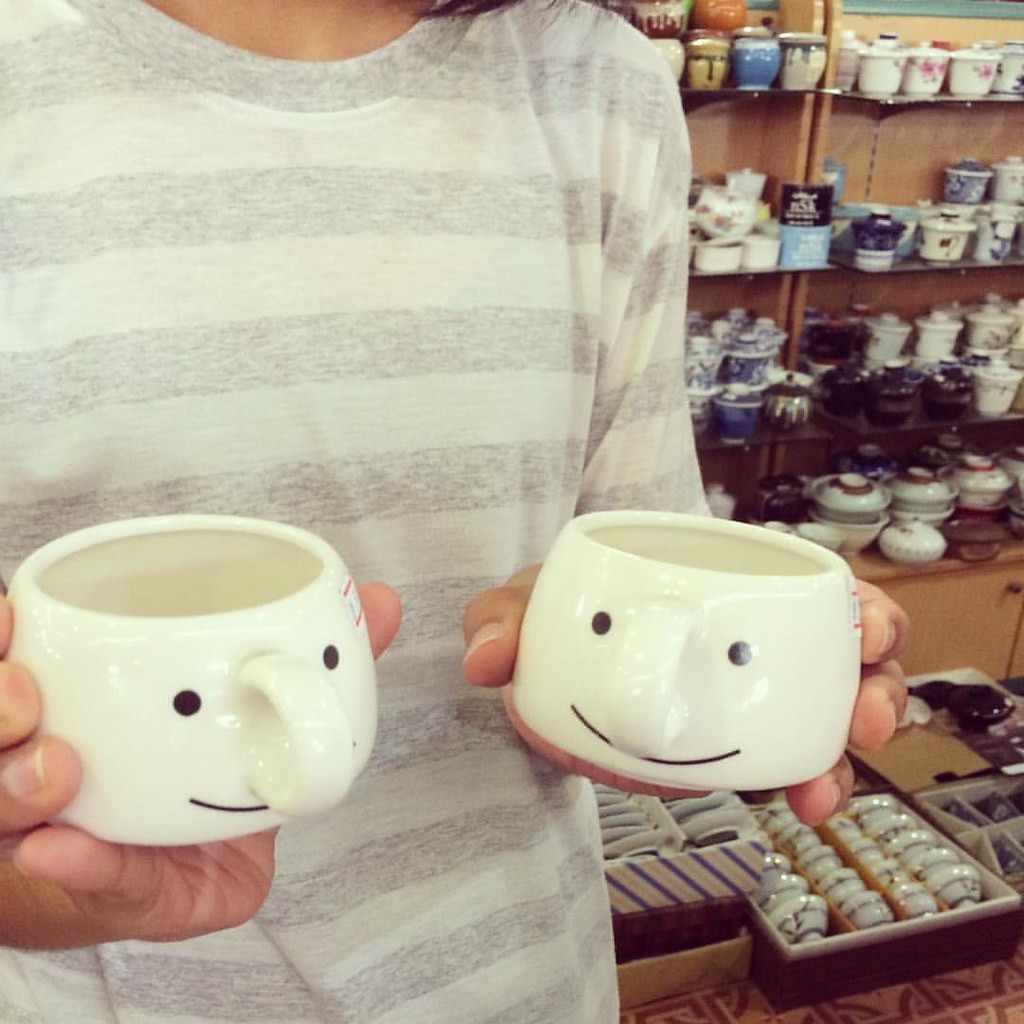In this detailed image, a woman with short brown hair, clad in a grey and white horizontally striped shirt, stands in a china shop, holding two small white teacups. Both teacups feature whimsical faces with black smiley mouths and handles positioned to resemble noses, with black dots above the handles for eyes. Behind her, the shelves are adorned with a wide assortment of teapots, vases, and an additional collection of teacups similar to the ones she's holding. The shelves also house boxes filled with matching sets of cups and teacups, each box displaying different patterns. The scene captures the inviting charm of the shop filled with meticulously arranged rows of delicate china and teacups.